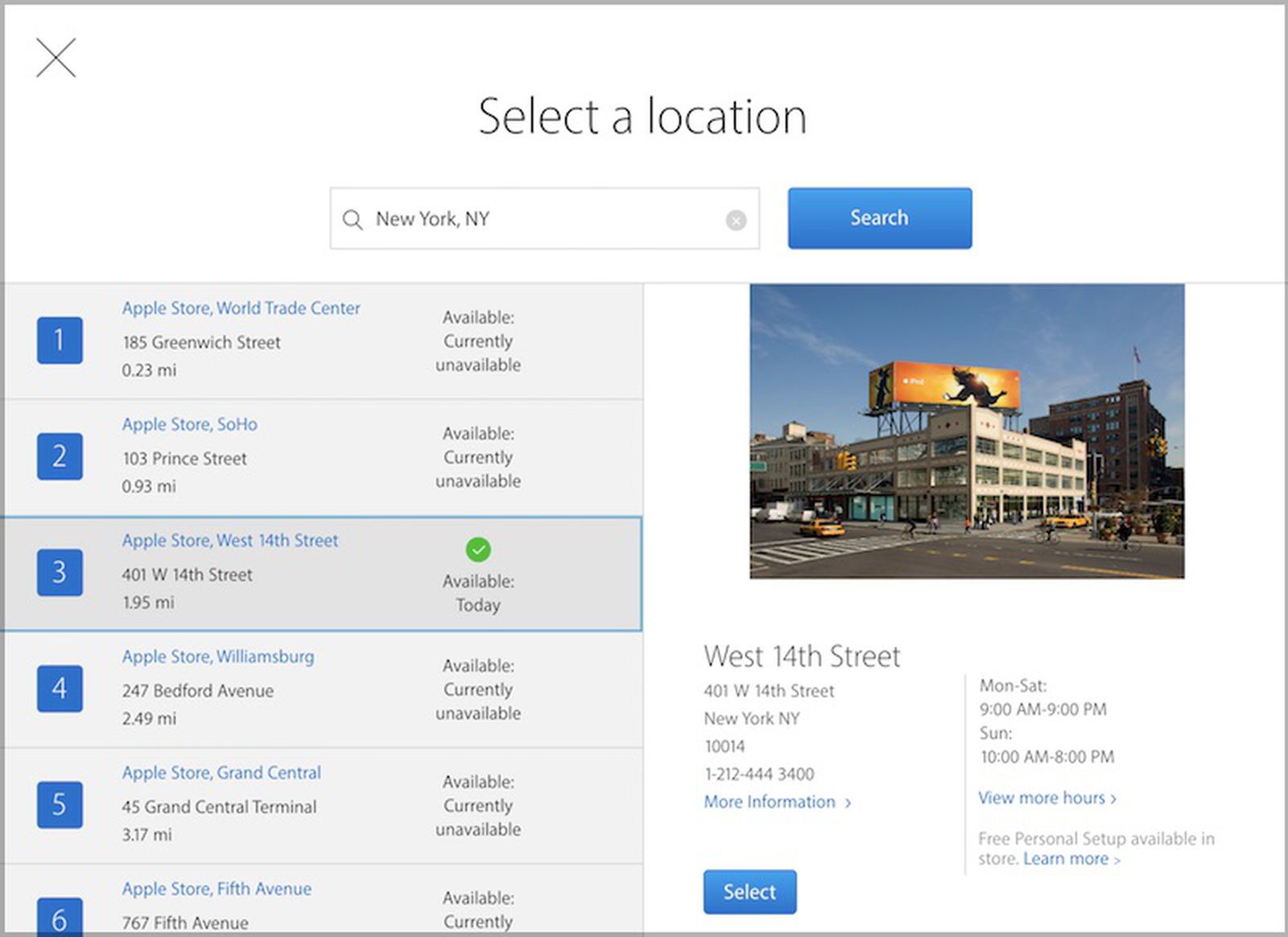This is a screenshot showcasing a website that lists various Apple stores. Prominently displayed at the top center is a title that reads "Select a Location." Directly below this, there's a search bar with the text "New York, New York," accompanied on the right by a blue "Search" button. Beneath this section, the left side features six Apple store listings. Each listing begins with a blue square number box. Next to the box, the Apple store's name or location appears in blue text at the top, followed by the store's address, and further below, the distance from the designated location. To the right of these details, the availability status of each store is displayed, indicating "Available," "Currently Unavailable," or "Available Today," with a corresponding green checkmark as applicable. The third listing stands out, being highlighted and circled by a blue box, suggesting it is the selected or recommended store option.